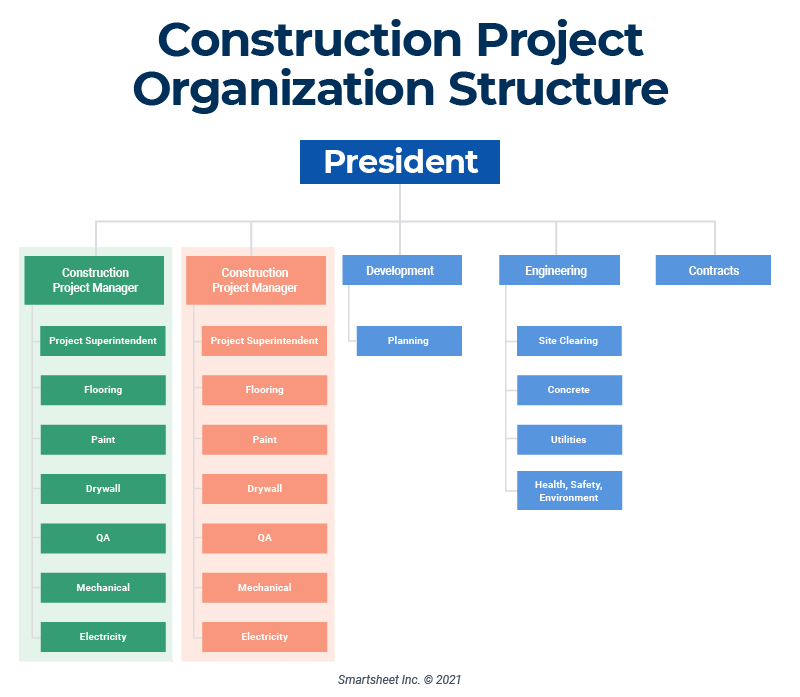This detailed and comprehensive infographic, set against a white background, is a horizontal flowchart depicting a "Construction Project Organization Structure." At the top, the title "Construction Project Organization Structure" is prominently displayed in black, while a blue rectangle directly below it is labeled "President" in white letters. Emanating from this "President" rectangle, a vertical blue line meets a horizontal blue line that branches into distinct columns, each represented by rectangles in various colors.

On the far left, the first column starts with a green rectangle labeled "Construction Project Manager," which cascades into several boxes beneath it: "Project Superintendent," "Flooring," "Paint," "Drywall," "QA," "Mechanical," and "Electricity." The second column is similar but differentiated by an orange color, also labeled "Construction Project Manager," followed by identical subdivisions as the first.

In the center, a blue column is designated for "Development" with a single box underneath marked "Planning." Continuing right, another blue column labeled "Engineering" features subdivisions for "Site Clearing," "Concrete," "Utilities," "Health," "Safety," and "Environment." Finally, on the far right, a blue column is labeled "Contracts."

Concluding the flowchart, the bottom of the image holds a copyright statement in black text, "Smartsheet Inc. Copyright 2021."

By encompassing these elements, the infographic provides a structured and detailed representation of the various roles and responsibilities within a construction project organization.